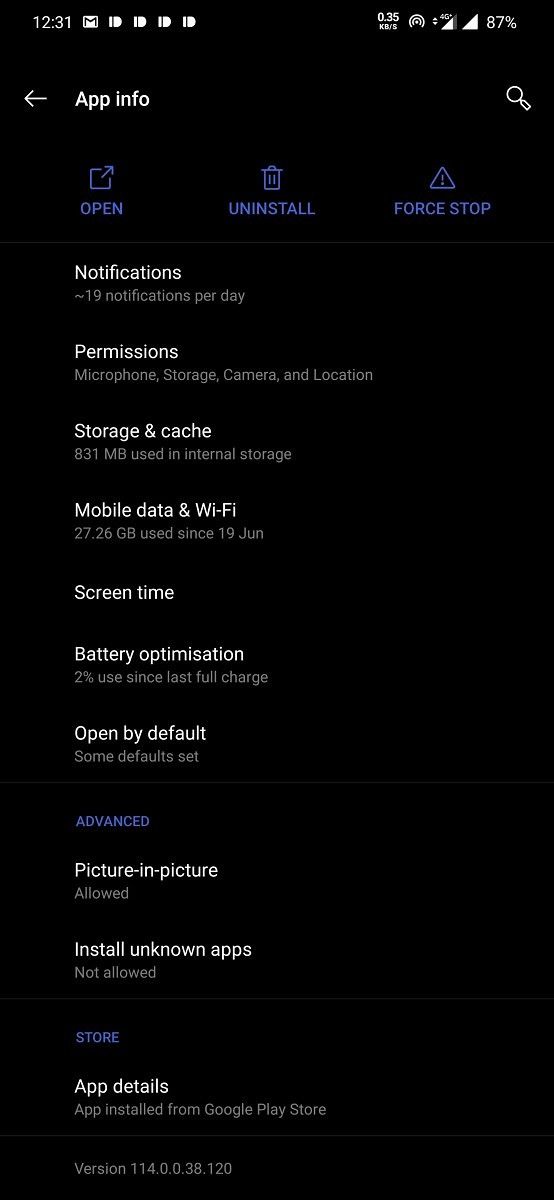A detailed screenshot of the 'App Info' page on an Android phone. At the top of the screen, the status bar displays typical Android notifications. Central to the screenshot are interaction options for the specific app: "Open" (indicated by an open icon), "Uninstall" (indicated by a trash can icon), and "Force Stop" (indicated by a triangle with an exclamation mark inside it).

Below these options, various sections provide detailed information about the app:
- **Notifications**: Displays "Approximately 19 notifications per day".
- **Permissions**: Lists permissions including Microphone, Storage, Camera, and Location.
- **Storage and Cache**: Specifies "831 MB used in internal storage".
- **Mobile Data and Wi-Fi**: Indicates "27.26 GB used since 19 June".
- **Screen Time**: Details the app's screen time usage.
- **Battery Optimization**: Notes "2% use since last full charge".
- **Open by Default**: Displays default settings, which are not specified.
- **Advanced**: Labeled in purple text, likely leading to more options.
- **Picture-in-Picture**: States "Allowed".
- **Install Unknown Apps**: States "Not Allowed".
- **Store App Details**: Another heading in purple indicates the app is "Installed from Google Play Store" along with version information.

Overall, the screenshot provides a comprehensive overview of the app's various settings and usage metrics on an Android device.